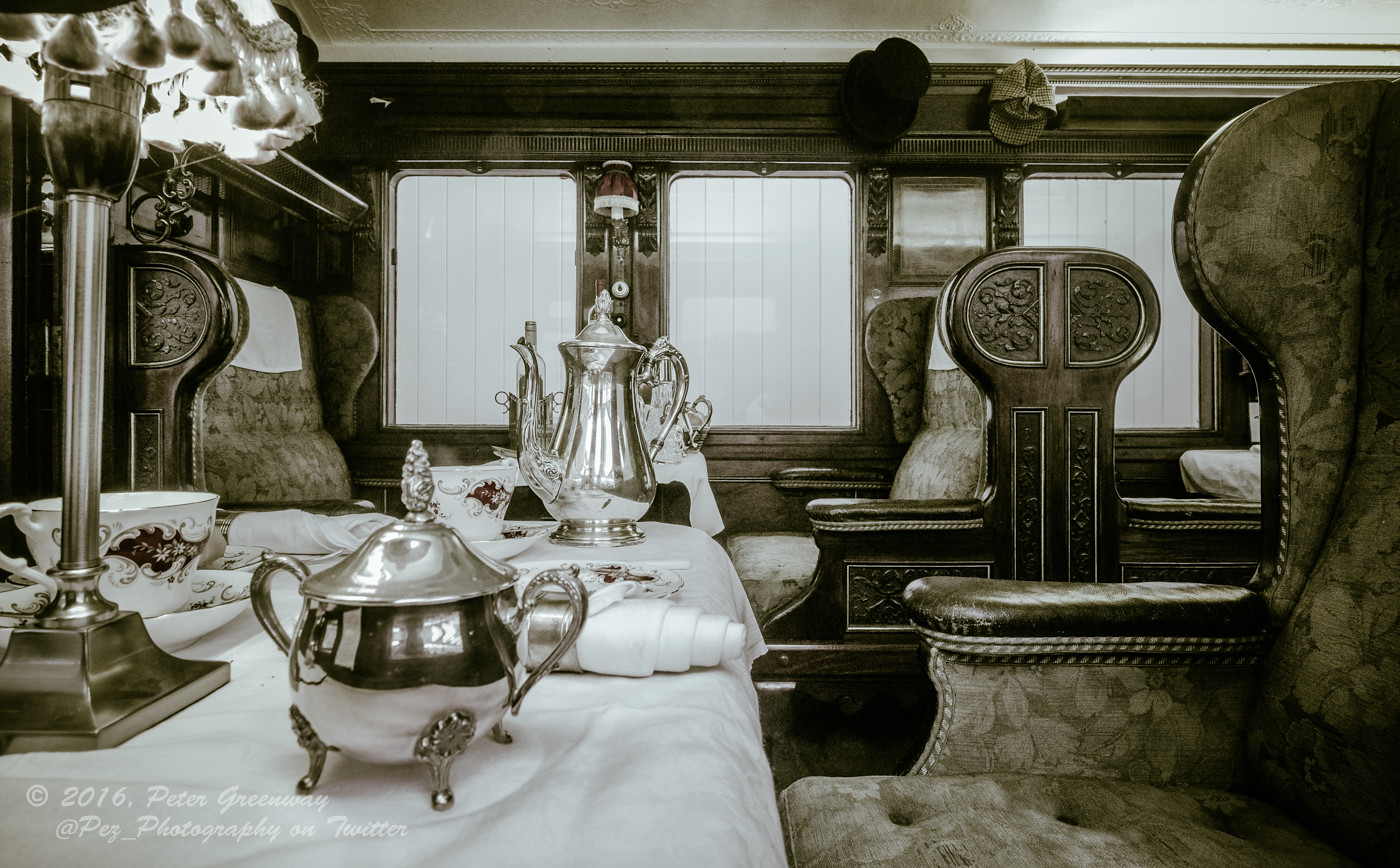This is a sepia-toned photograph capturing the interior of a luxury train car, evocative of the 1800s. The cabin is adorned with elegantly draped white linen tablecloths set with exquisite china, including teacups, saucers, and ornate silver teapots. A black top hat and a plaid hat hang from the intricately carved wooden paneling of the train. The scene is well-lit by a lamp with a metallic base and fringe, casting a warm glow over the sumptuous setup. Rolled napkins with silver holders add to the opulent atmosphere. In the photograph, there are numerous booths with tables nestled between plush seats, framed by a series of windows that line the far side of the car. The lower left-hand corner of the image is marked with the text "February 2016, Peter Greenway" along with a Twitter handle, suggesting the image was captured by modern photographer Peter Greenway.